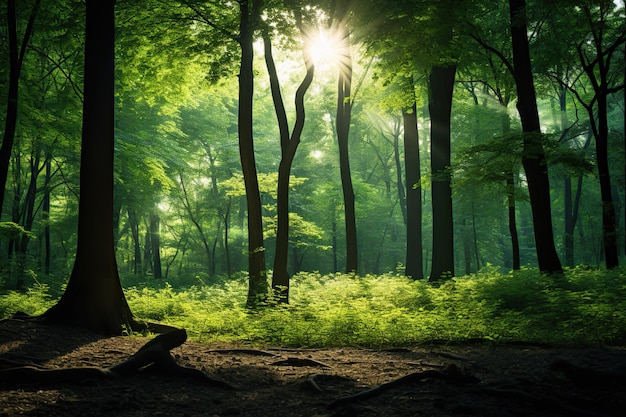This detailed image depicts a serene and lush forest, characterized by tall trees with dark, blackish trunks due to the limited sunlight filtering through the dense canopy. The foreground reveals a dirt trail running from right to left, with roots protruding and a tree emerging from the ground on the left side. Approximately one-third up from the bottom, the forest floor is adorned with a variety of green underbrush and foliage. In the middle of the image, where the forest becomes denser, the sunlight breaks through the leaves or an opening in the canopy, creating a bright, illuminating focal point that barely lights up the surrounding trees. The sun creates a noticeable lens flare, adding to the peaceful, almost mystical ambiance of the scene. This area is populated with numerous trees, some prominently visible in the foreground and countless more fading into the background, all contributing to the rich verdant landscape.